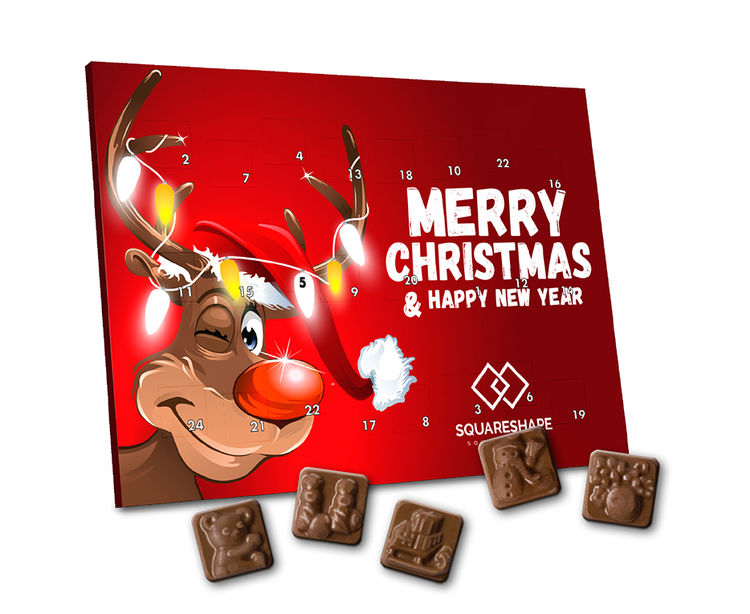This image features a vibrant red advent calendar designed for the 24-day countdown to Christmas. The calendar is adorned with numbered spaces from 1 to 24, each hiding a piece of chocolate behind it. These chocolates each bear festive designs, such as a bear, a snowman, and a sled. Dominating the left side of the calendar is an animated reindeer, likely Rudolph, characterized by his glowing red nose, a winking eye, and a Santa hat that drapes down. His antlers are festively decorated with stringed Christmas lights. The right side of the advent calendar is marked with bold white letters proclaiming "Merry Christmas," and beneath it, "Happy New Year." At the base, five pieces of chocolate are visibly showcased, hinting at the daily treat awaiting each day in December. The calendar is produced by the brand Squareshape, aiming to bring a sweet and whimsical touch to the holiday season.